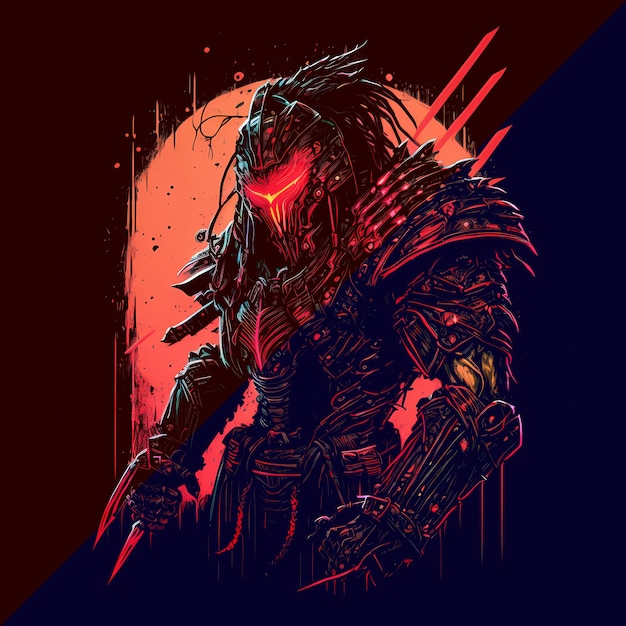The image depicts a comic book-style figure exuding a menacing presence, resembling a formidable boss character from a video game. The central figure is an alien warrior clad in intimidating, full-body armor that is predominantly black with intricate red lines illuminating its face mask and other details. This warrior, which evokes a sense of diabolic power, is equipped with claw-like gloves featuring blade-like spikes, reminiscent of Wolverine. The background of the image is split diagonally, with the top half in dark brown and the bottom half in a very dark blue. An orange, sun-like orb with a shredded line design radiates behind the warrior, casting an eerie glow. The overall composition, akin to a dramatic poster, highlights the alien warrior's readiness for battle, standing defiantly against the contrasting backdrop.